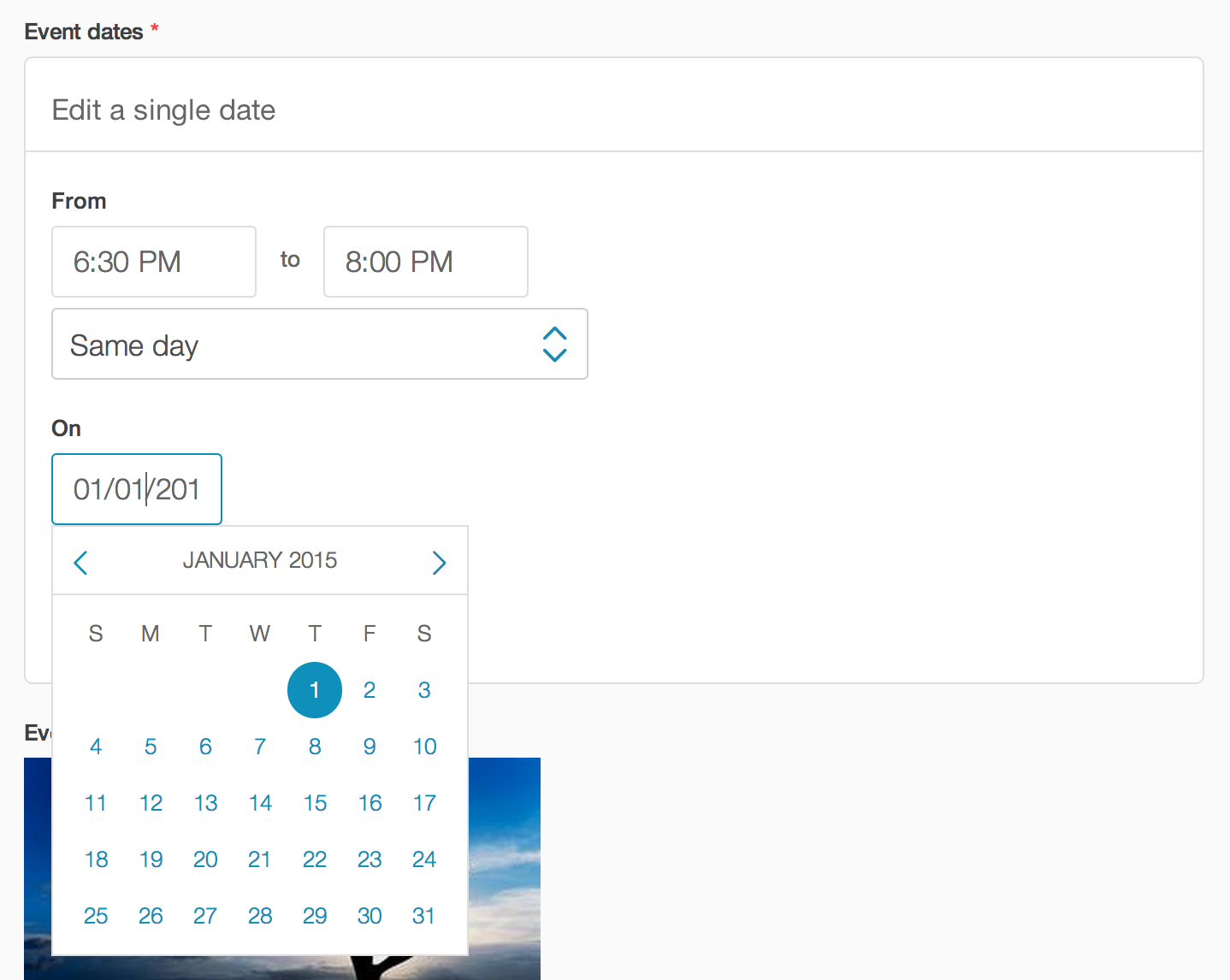The image features a calendar section for an event scheduled on January 1, 2015. At the top, the text "Event Dates" is prominently displayed in bold, black font with a red asterisk beside it, though the significance of the asterisk is unclear. Below, there is a section labeled "Edit a Single Date," detailing the event time from 6:30 PM to 8:00 PM on the specified day. A January 2015 calendar occupies approximately 75% of the image, making it the central focus. In the background, a partial view of a picture with a blue sky and scattered clouds is faintly visible, though largely obscured by the calendar overlay. The overall layout appears straightforward but lacks additional context or explanations.